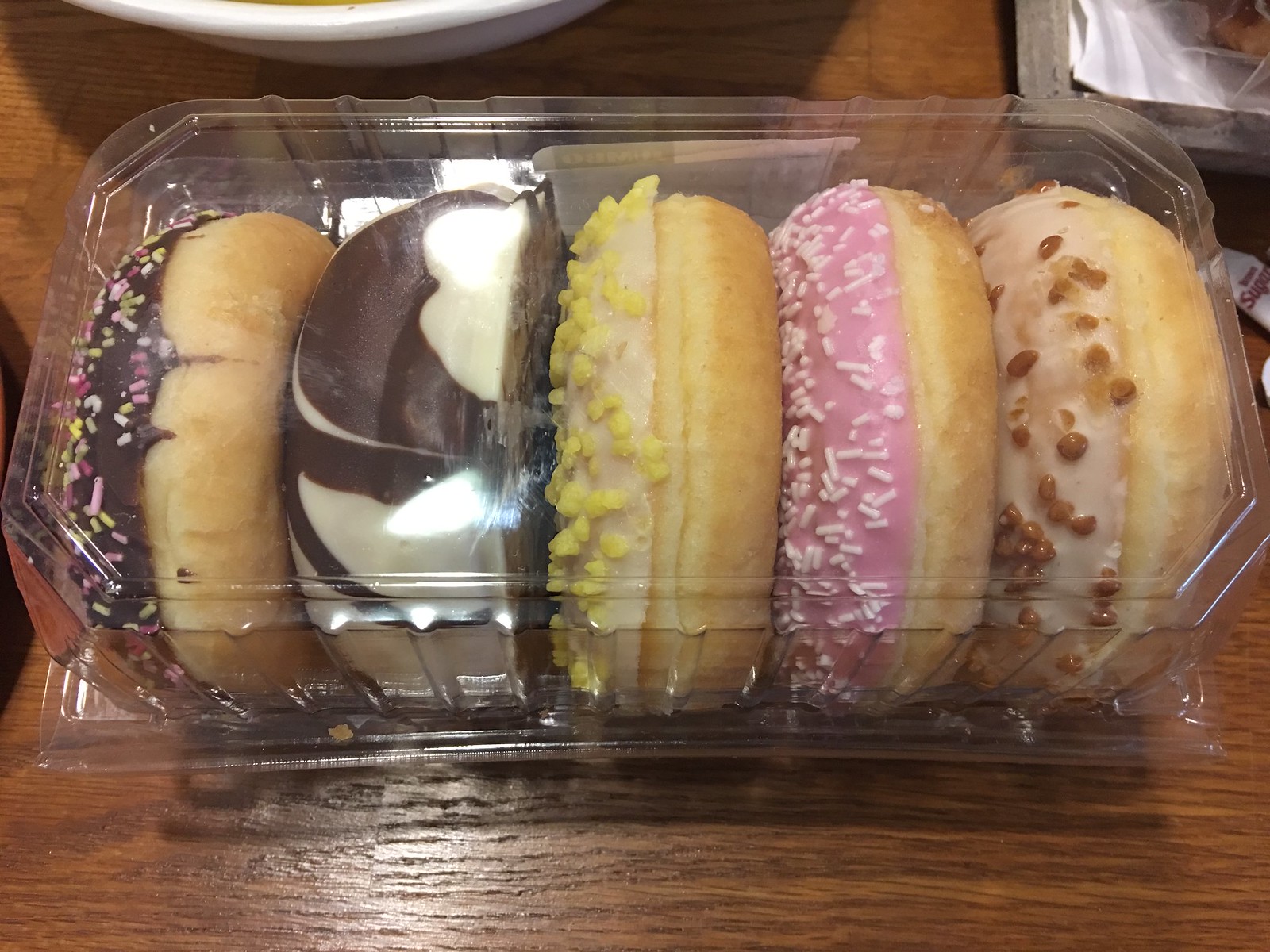The image showcases a close-up of five beautifully decorated donuts arranged vertically in a plastic container, placed on a wooden surface. Each donut displays a unique array of colors and toppings: one with chocolate icing adorned with multi-colored sprinkles, another featuring a combination of white and dark chocolate frosting, a third with vanilla icing and yellow sprinkles, a pink frosted donut with white sprinkles, and the last one with white icing topped with brown sprinkles that resemble caramel or crunchy chocolate pieces. The photo captures the vivid details of the donuts, emphasizing their varied textures and flavors.